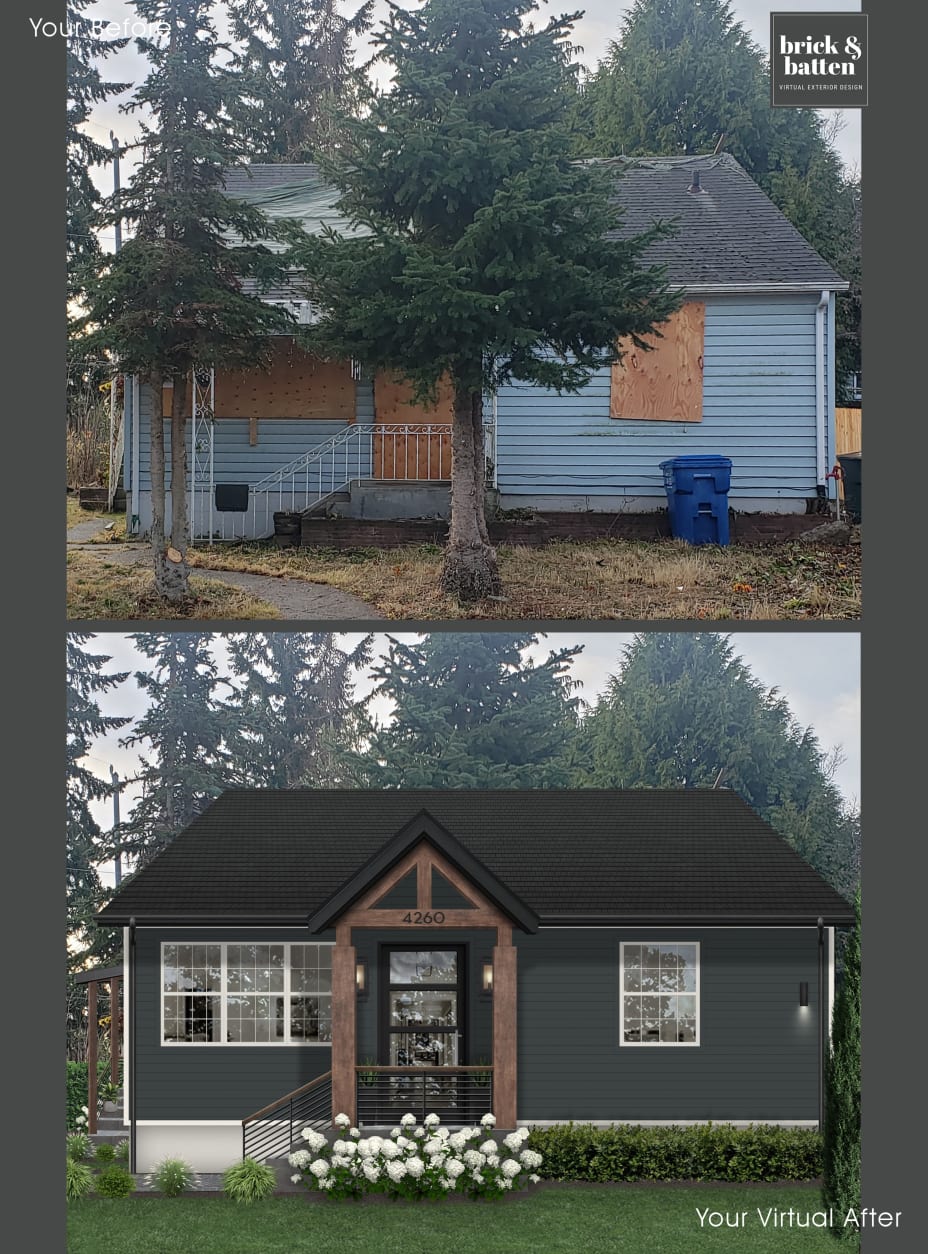The image is a split "before and after" comparison of a house, presented on a solid dark gray background. The top section shows a run-down, light blue house with boarded-up windows, a white handrail, and a beaten-up roof. The yard is overrun with weeds and sparse grass, and there is a blue recycling bin and a garbage can in front. The surroundings include a couple of large trees.

In contrast, the bottom section features a digitally-rendered makeover of the same house, labeled as a "virtual after" by the company Brick & Batten. This virtual renovation transforms the house with a new, gray exterior and a brown arch over the door. The white handrail has been replaced by a brown one, and the front yard is now adorned with white flowers and shrubs. The grass appears lush and well-maintained. The same background trees anchor both images, emphasizing the transformed look of the house and yard.